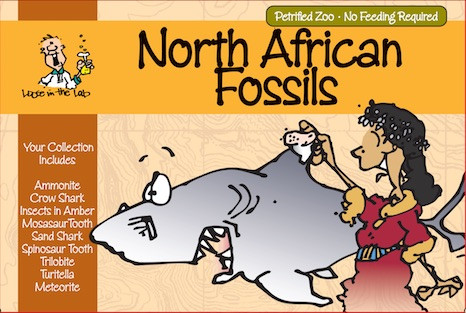In this cartoon-style advertisement, set against an outdoor backdrop, a striking illustration captures a woman and a shark. The woman, with long black hair and a floral crown, dons a red dress accented by a tan and blue belt. Her pointy nose and the tan, fluffy trim on her sleeves and collar add to her distinct appearance. She holds a white object aloft in her arm, her expression directed towards the left. Beside her, the menacing figure of a gray shark looms, his dark-to-light gradient body, bulging white eyes with drawn eyebrows, and gaping mouth filled with sharp teeth enhance his intimidating presence. The top of the image reads "Petrified Zoo, No Feeding Required, North African Fossils." On the left, a list details the fossil collection available: Ammonite, Crow Shark, Insects in Amber, Mosasaur Tooth, Sand Shark, Spinosaurus Tooth, Trilobite, Turritella, and Meteorite. Additionally, a graphic of a man in a white shirt holding a bottle is captioned "Loosen the Lab." The entire setup suggests it might be the top of a fossil collection box for sale.